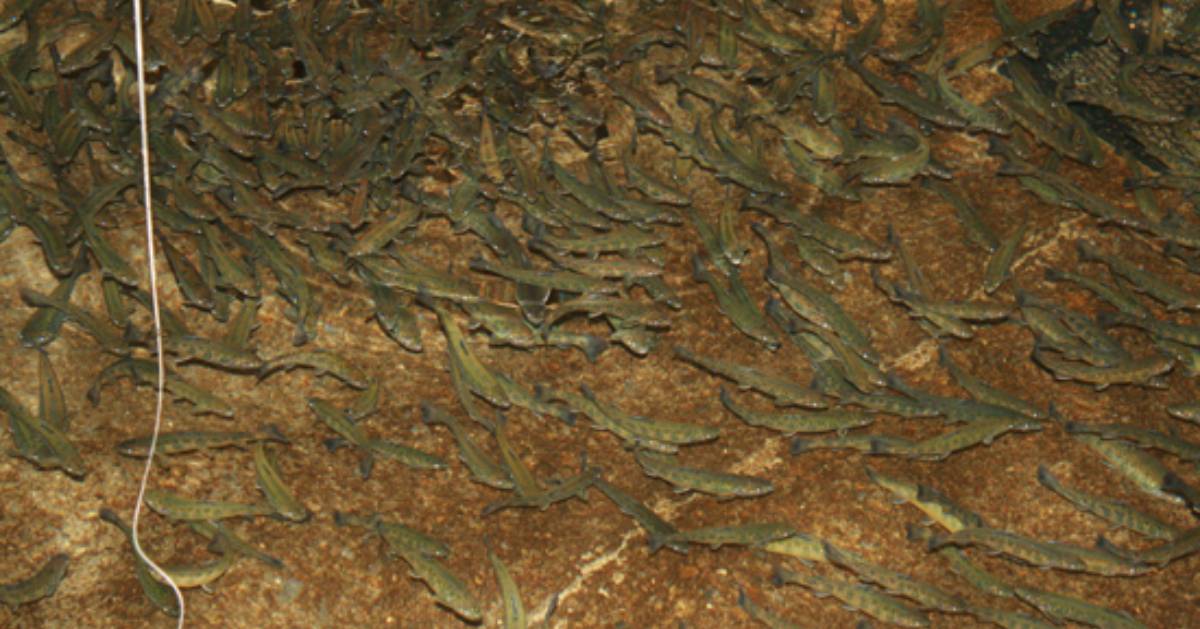The photograph appears to be taken either outdoors or in a fish enclosure and depicts hundreds of green-colored fish swimming together, predominantly bunched up in the top left area. These fish, which have yellow bellies beneath their green upper layers, are scattered throughout the photo, becoming more spread out towards the edges. They swim above a brown rock-patterned surface, suggesting a shallow pool or body of water. The background is a mix of rusted brown, beige, and white hues. A white string or thin rope descends from the top left and curls slightly at the bottom. Additionally, in the top right corner, there is a black metal grate that the fish appear to be swimming over.